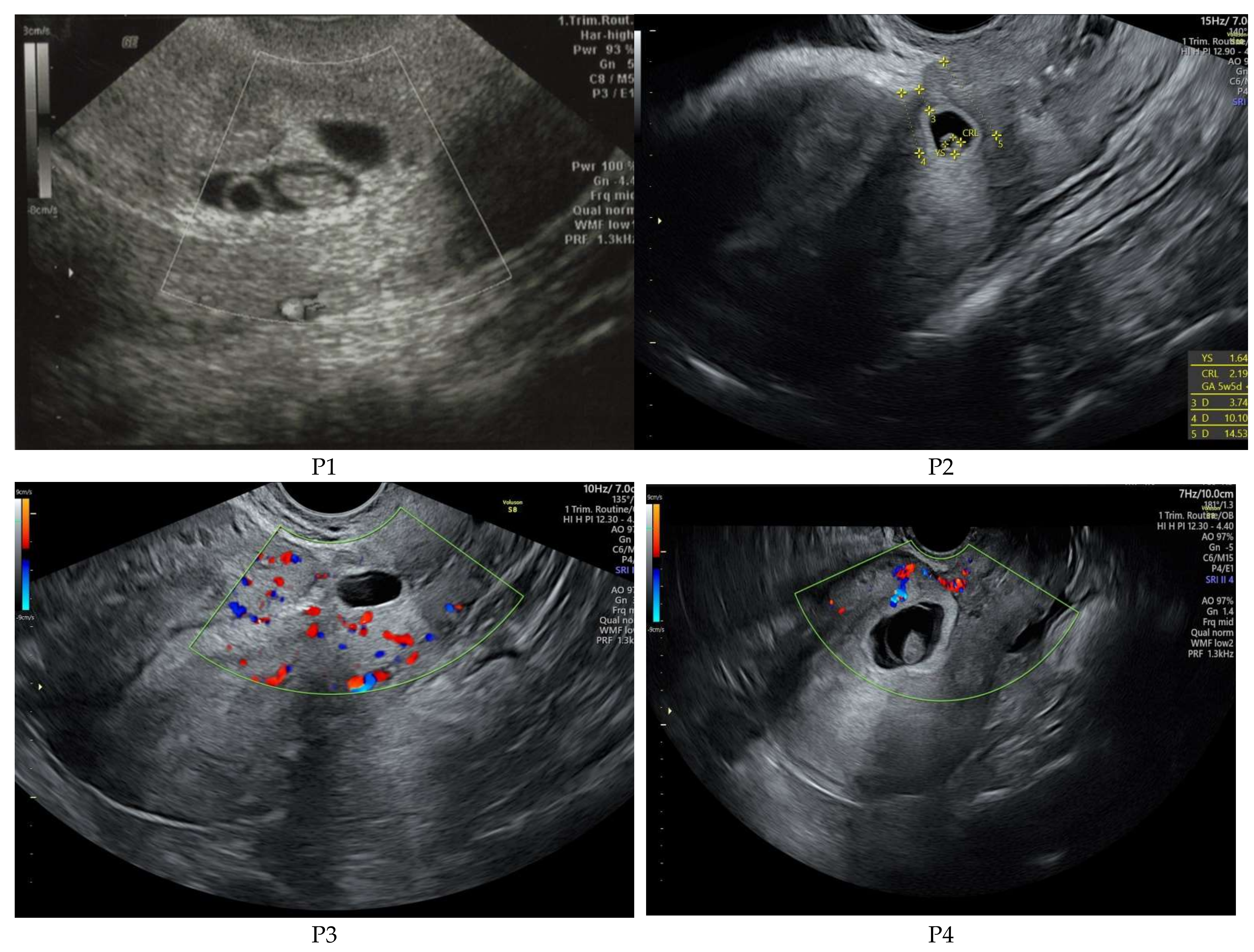The illustration features a set of four ultrasound images arranged in a 2x2 grid and labeled P1, P2, P3, and P4, each image being square-shaped or rectangular. The ultrasounds showcase different sections or angles of the scanned area. The top-left image, P1, displays a gray shaded area with accompanying technical information on the right. The top-right image, P2, has a darker gray background with some yellow cross markers near the top and more textual data on the right side. The bottom-left image, P3, features a predominantly gray area highlighted by bright red, blue, and light blue splotches in the center, alongside a color scale on the left. The bottom-right image, P4, is similar to P3, with colorful splotches in the middle indicating various heat sensitivities—red for hotter areas and blue for cooler areas. Each image has a focal point that appears like a hole or tear, with the exact subject matter remaining unclear.